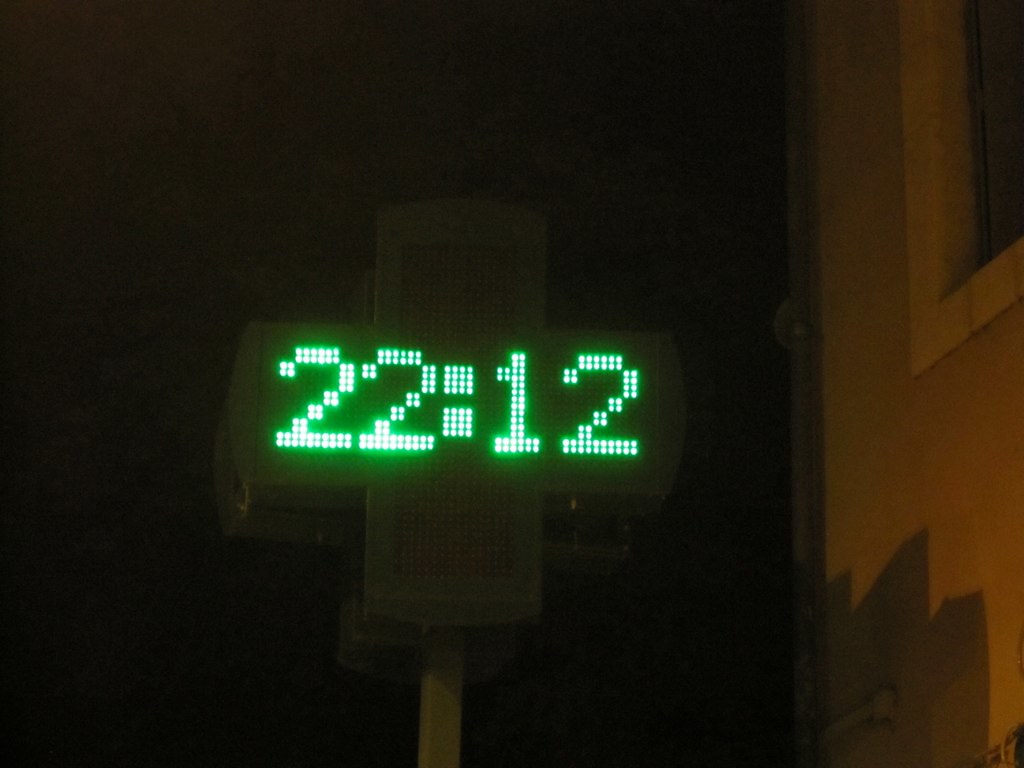The image is a horizontally oriented photograph depicting a large, digital clock in the shape of a cross. The photograph appears to be taken outdoors at night, indicated by the almost completely dark background reminiscent of the night sky. The clock, mostly black with a dark green border, displays the time as 22:12 in bright green LED digits. A thick, silver metal pole supports the clock. To the right of the clock, a building is partially visible, illuminated by a light that casts orange hues and shadows on its surface. The lower half of the building shows a darker shadow, and a window with white trim is faintly seen. The overall scene is very dark, with no other visible text or details in the image, emphasizing the glowing clock and the shadowy outlines of the adjacent building.